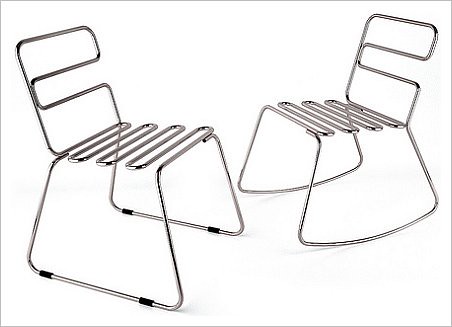In this detailed color image, two custom-made kitchen chairs are prominently displayed against a stark white background, bordered by a thin black square. Both chairs are crafted entirely from shiny, silver chrome metal, featuring a unique spiral or paperclip design. The seat of each chair is formed by thick, round wires that interweave in squiggly lines, providing a comfortable seating surface. The backrest of the chairs is composed of the same chrome wire, forming a rectangular outline with an additional squiggly line down the center. The chair on the left is stationary, identifiable by its four small black rubber cushions at the bottom of its legs. In contrast, the chair on the right is a rocking chair, characterized by its arched base that allows it to rock back and forth. The intricate and mirrored design of the chairs adds an artistic touch, making them both functional and visually compelling.